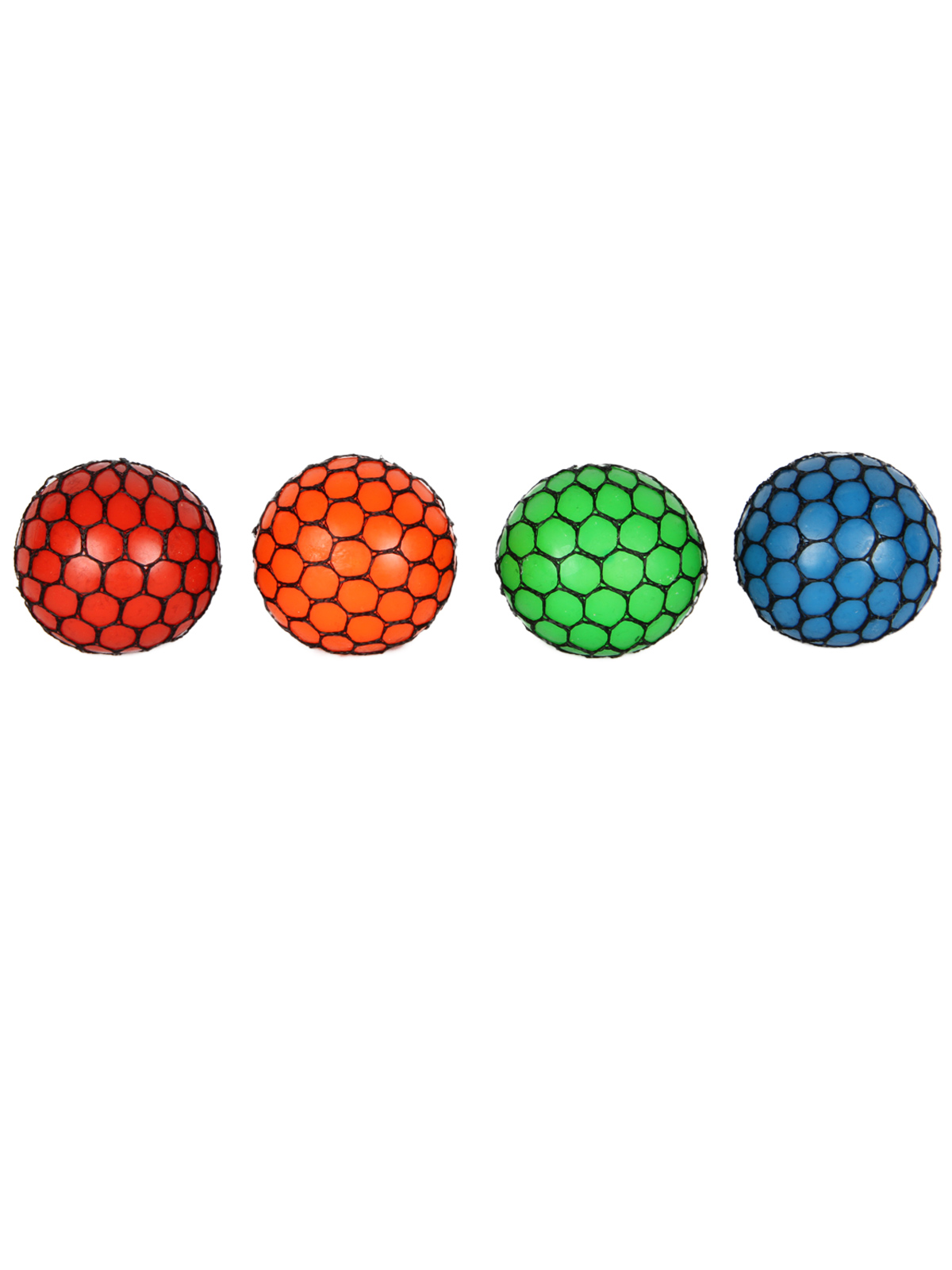In a minimalist photograph set against a completely white background, four round objects resembling bouncy balls are meticulously arranged in a straight horizontal line. Each of these spheres is decorated with black lines forming hexagonal patterns, reminiscent of a soccer ball's design. The ball on the far left is a striking black adorned with red lines. To its right, the second ball is bright orange, also featuring the same black hexagonal lines. The third sphere is a vibrant shade of green, just a tad darker than lime green, again showcasing the characteristic black lines. Completing the lineup, the ball on the far right is a deep blue, maintaining the consistent pattern of black lines. The vivid primary colors of red, orange, green, and blue, contrasted by the stark white background and the black hexagonal designs, create a visually compelling and balanced composition.